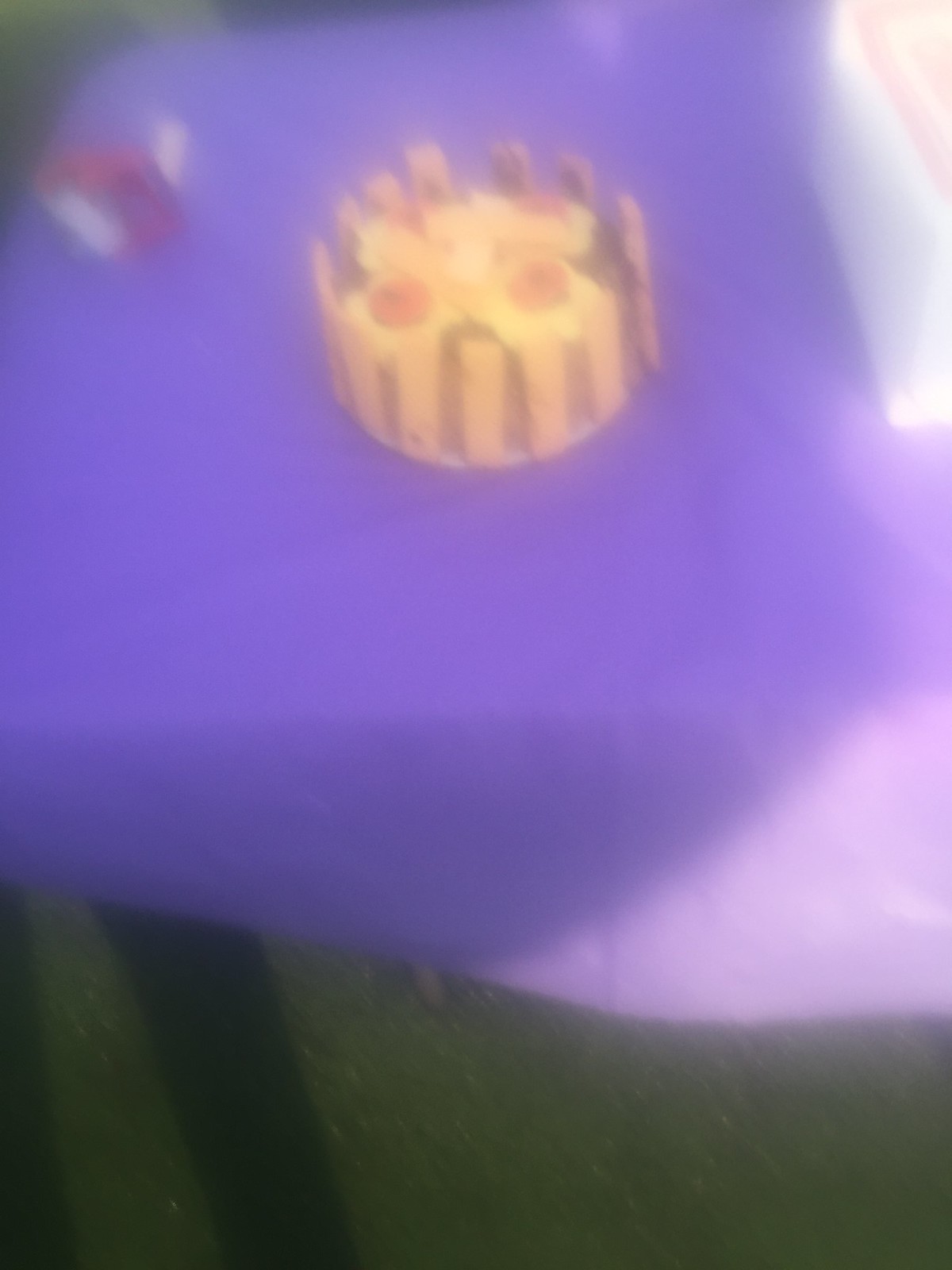The image is heavily blurred, presenting a challenging scene to interpret definitively. In the upper left-hand corner, a dark gray curve begins thinly on the left and arches upward towards the center, lightening slightly at the top center-left. The upper right-hand corner features a white shape that starts at the very top right center and transitions into a pale pink that curls around, with the central part being almost white and the outer edges a thicker white. This shape extends downward, curving down to the right, finishing with a pointed end.

Imagining the scene, it could be perceived as a tree trunk stretching from left to right across the frame. Just next to where this trunk becomes visible in the top left, there appears to be a floating white object adorned with a red scarf-like feature.

Central to the image is a peculiar object resembling a yellow cake, with seven sticks protruding from its sides. This object also has two orange spots in its middle, and four brown marks positioned at the front. From the bottom left to the bottom right of the frame, there is a wavelike formation of dark green, adding an additional layer of indistinct texture to the scene.